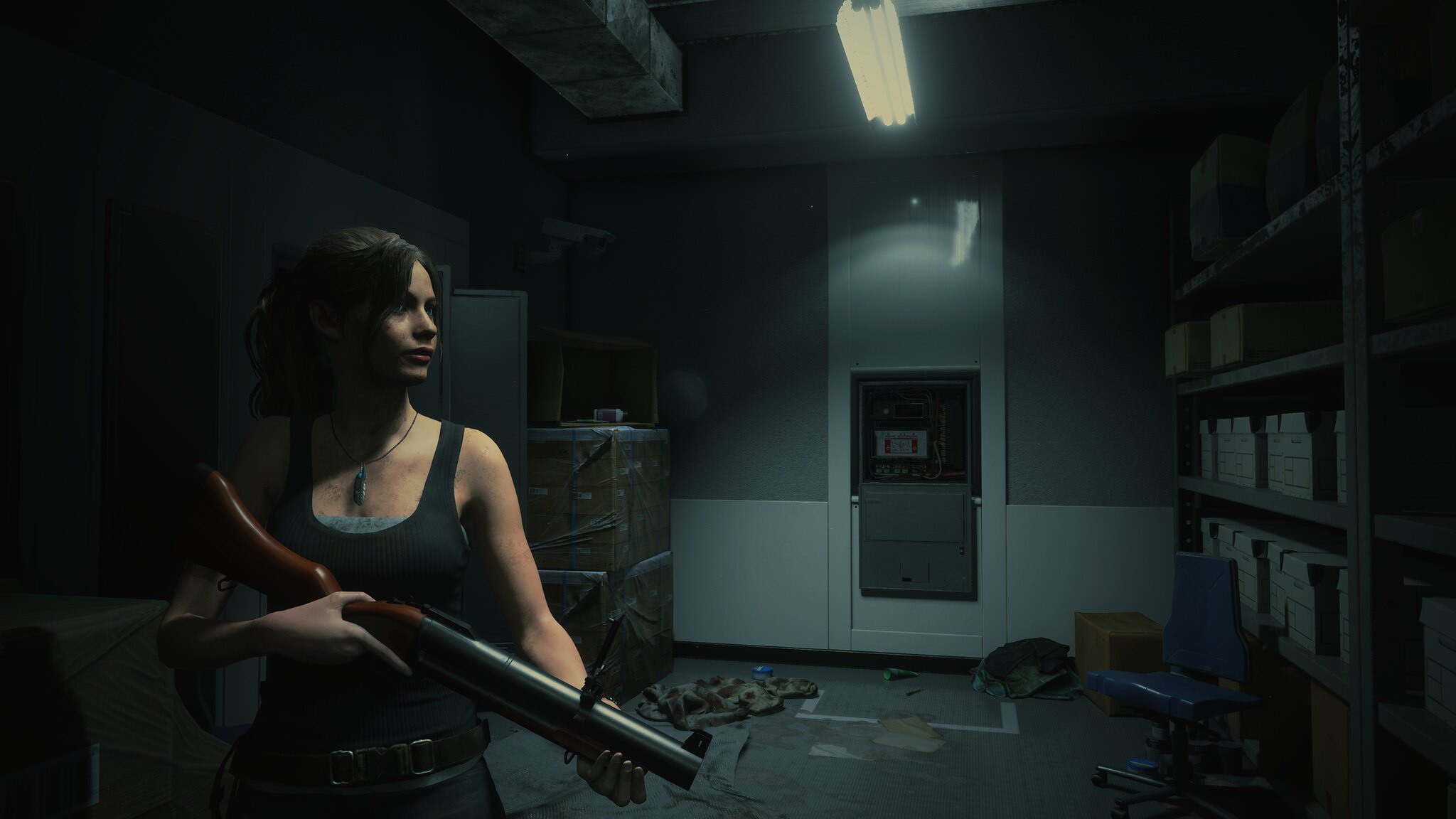The color photograph from a video game portrays a young woman, likely in her twenties, standing in the left third of a horizontal, rectangular frame. She exudes strength with her muscular build and is dressed in a dark-colored tank top over a gray tube top. Her outfit is completed with a black leather belt with a square buckle and dark pants. Around her neck, she wears a leather lace with a pendant hanging from it. Her hair is long and brown, tied up, revealing her intense focus as she gazes across her left shoulder. In her hands, she grasps a sawed-off shotgun with a wooden handle, which appears futuristic.

The setting is a cluttered, disarrayed office building, resembling a storage room, evident from the metal shelves filled with document boxes and a yellow and light blue swivel office chair positioned in front. Cardboard boxes and rubbish are scattered on the floor, contributing to the chaotic ambiance. A gray cabinet with open doors stands alongside the shelves. High above, a fluorescent light casts a dim glow, insufficiently lighting the room, adding to the sense of anticipation and readiness for action. Reflections in the back suggest the presence of an electrical system mains, enhancing the gritty, enclosed atmosphere of this modern gaming scene, with hints resembling the aesthetic of the Tomb Raider game series.